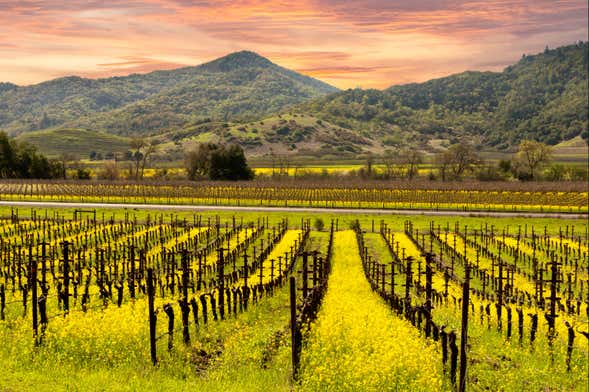This photograph captures a vineyard during an off-season, with rows of tall brown wooden posts and horizontal strings typically used to support grapevines, now void of any vines. The vineyard is overtaken by yellow and green wildflowers, creating a lush, almost overgrown appearance. The foreground shows a hill sloping down towards the center of the image, with these posts arranged in long, vertical rows. Cutting through the middle of the photograph is a narrow, gray road, possibly asphalt, dissecting the vineyard. Beyond the road, the landscape mirrors the foreground, featuring more rows of posts standing in verdant greenery. In the background, a range of mountains rises, adorned with dark green trees and some barren patches with indistinct structures. The sky above is a dramatic spectrum of rich oranges, purples, and grays, suggesting either a sunset or twilight, casting a warm glow over the serene, countryside scene.